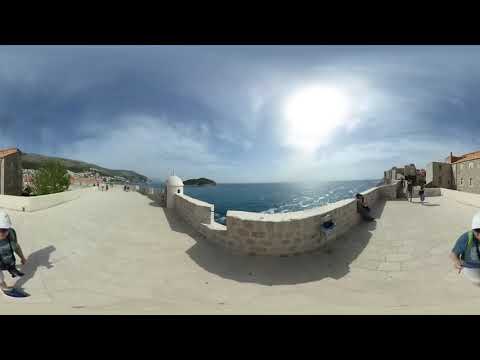The photo depicts a scenic seaside view taken from a slightly warped, wide-angle perspective, which introduces some curvature to the landscape. In the foreground, a lime-colored, brick-like stone pathway or roadway runs parallel to the coastline, divided by a series of stone barriers or fences that separate the path from the ocean. This pathway appears somewhat rocky and uneven, creating a rustic feel. The ocean, bright in the sunlight, reflects the sun's rays back into the sky. On both the left and the right sides of the image, there are buildings visible in the distance across the water. Additionally, on the right side, an island or a part of a peninsula is visible, hinting at a landmass further away, though it is not clearly connected to the main land due to the distance. The sky is vividly blue with wispy clouds scattered across, adding to the serene atmosphere. People are seen walking along this path, but they are too blurry to make out any specific details. The overall scene exudes a calm, coastal charm.